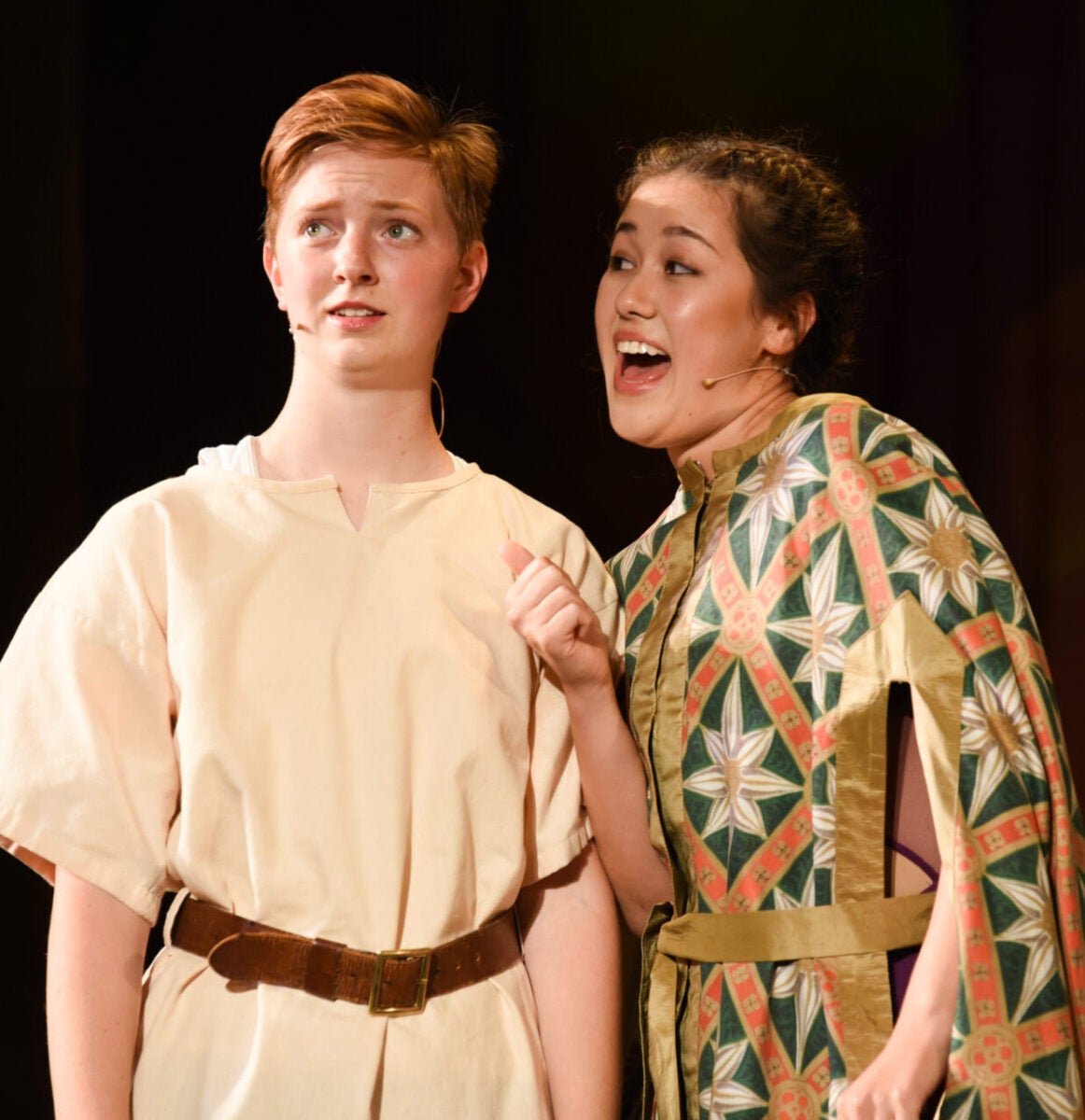This color photograph features two individuals, presumably engaged in a theatrical performance, as suggested by their headset microphones and expressive postures. The background is a stark black, making the subjects stand out prominently. On the left is an individual with indeterminate gender, characterized by short, oblong, red hair and wearing a light tan tunic, cinched at the waist with a brown leather belt. This person is slightly turning away and has their mouth open, possibly singing or speaking loudly.

To the right is a female with long, brown hair intricately braided into two French braids. She has striking brown eyes and is adorned in a vivid, floral-patterned garment that features a crisscrossed ribbon design with colors including red, green, white, brown, gold, and peach. Her mouth is wide open, revealing her white teeth, as she gazes in the direction of her companion, engaged intensely in the moment. Their dramatic attire and dynamic expressions strongly suggest that they are mid-performance in a play or theatrical production.